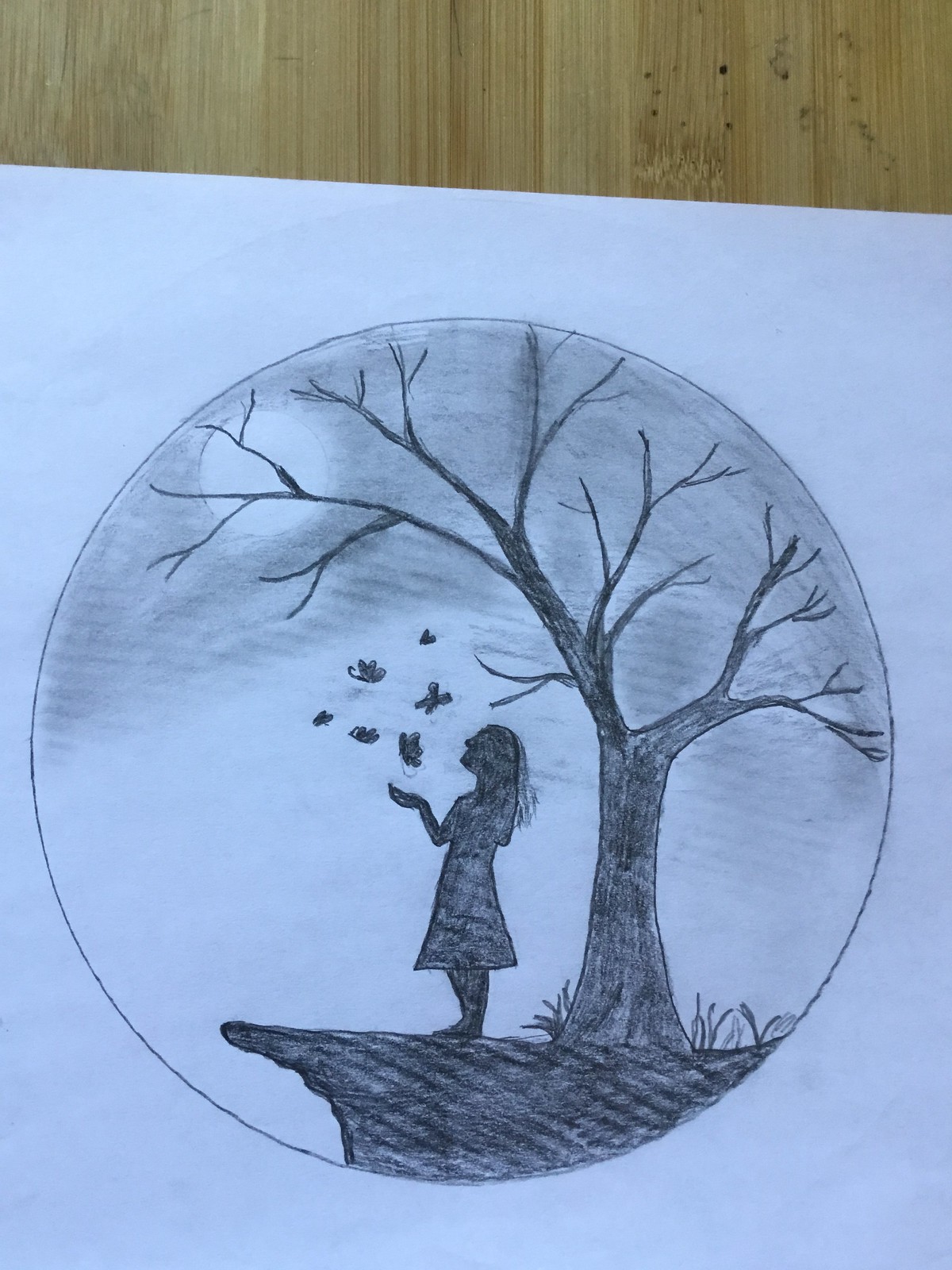This is a meticulously crafted pencil drawing on white paper, set against a background of light brown wood paneling. The paneling is visible at the very top of the image, providing a subtle, warm contrast to the artwork. The drawing is circular in form and showcases intricate shading and detail. 

At the heart of the illustration stands a tree with branches fanning out gracefully. Below it, a cliff, shaded in black, adds depth and texture to the composition. Standing in front of the tree is a figure, possibly a woman or child, depicted with long flowing hair and a dress that falls elegantly to the ground. Her hand is extended towards a cluster of butterflies, rendered as if caught mid-flight. 

In the background, partially obscured by the tree branches, is a luminous celestial body—either the moon or the sun—casting subtle light and contributing to the ethereal ambiance of the scene. The entire drawing is detailed and delicate, with a harmonious blend of natural elements and soft, artistic touches, capturing a moment of serene beauty and wonder.